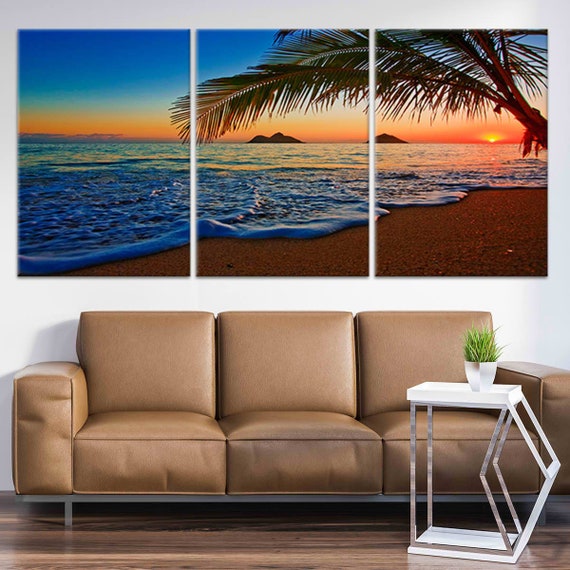The image is a full-color, square photograph taken indoors with artificial lighting, clearly staged to highlight an elegant interior setting. Dominating the scene is a large brown leather couch with thick, plush cushions giving it a luxurious feel. The couch is situated on a polished wooden floor. To the lower right of the image, there is an avant-garde table, constructed with a combination of metal and glass, with a small white planter on top that contains a green grass-like plant.

Directly in front of the couch is a coffee table with a distinct silver frame, adorned with only a single tray on top. The backdrop wall is a subtle off-white blue, creating a neutral canvas that enhances the featured artwork above the sofa. The highlight of the image is a series of three canvases mounted above the couch, which together form a cohesive beach scene. The artwork depicts a serene landscape with a beach in the bottom right, waves gently reaching the shore, and a palm tree arching into the scene from the center right. The sky transitions from orange near the horizon to a tranquil sky blue, capturing a picturesque sunset over the water, and includes an island in the distance. The overall composition suggests a carefully curated and artistic interior design.